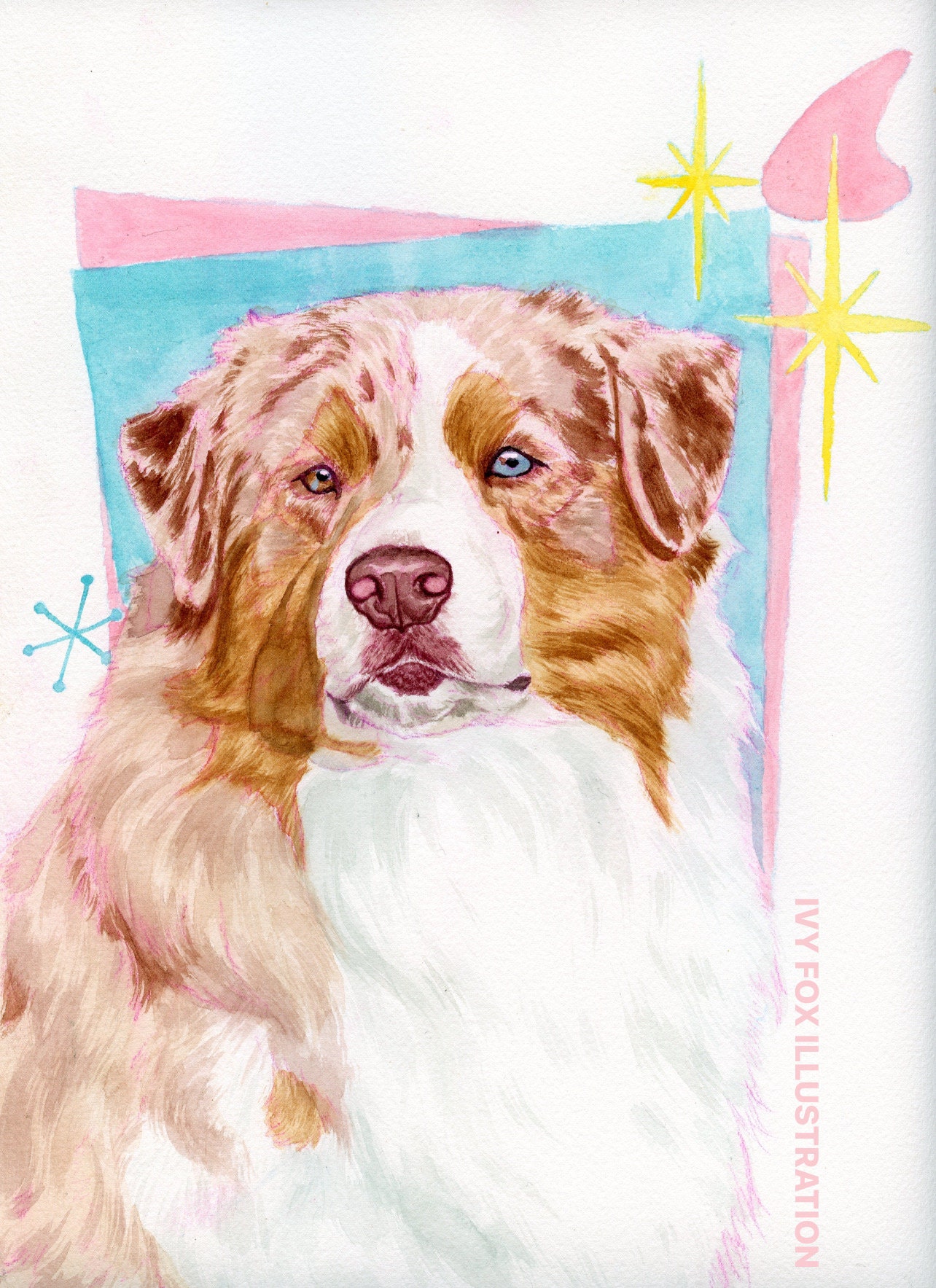This detailed illustrated drawing portrays a large dog with a mix of brown and white fur. The dog's eyes exhibit heterochromia, with one blue eye and one pink eye, and it also features a pink nose. The dog’s fluffy white fur is prominent on its chest, and its ears are floppy. Surrounding its head and forehead is the darkest brown fur, cascading into lighter auburn hues. The background combines a blue square overlapping a pink square, and there are yellow starbursts in the upper right corner and a large blue star shape on the left. In the lower right corner, pink text reading "Ivy Fox Illustration" is rotated 90 degrees on a white background. The image also includes a one-inch border on the right and a two-inch border at the top.